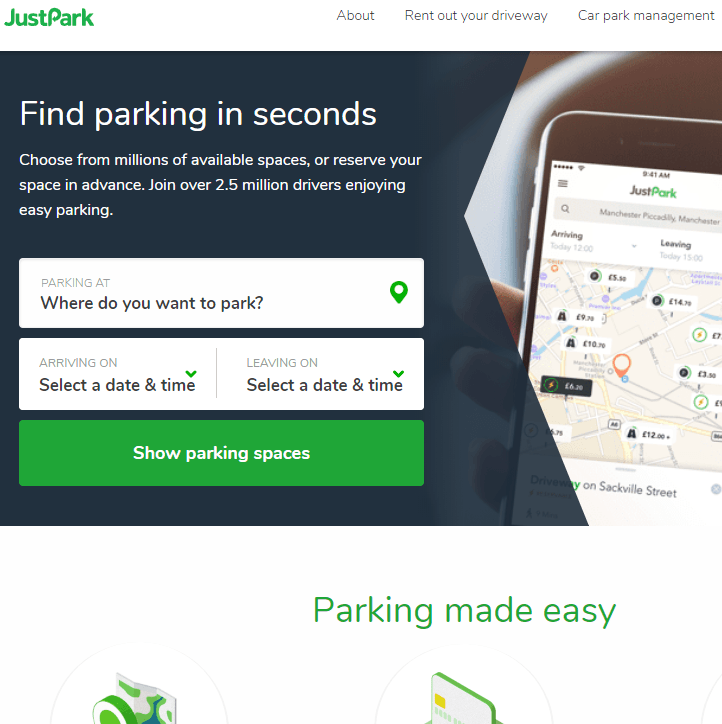**Image Description:**

The advertisement features a predominantly white and blue background with a green and black-text overlay. The top portion of the ad has a white background. On the left-hand side, green text reads "Just Parked," and black text within that segment says, "Right now it's your driveway, car park management."

Below this section, the background shifts to a unique shade of blue. On the upper left-hand side, bold white text promises, "Find parking in seconds." It further elaborates in white text, "Choose from millions of available spaces, or reserve your space in advance. Join over 2.5 million drivers and enjoy easy parking."

Towards the middle, a white rectangular box with gray text prompts users with, "Parking at," followed by a black text placeholder, "Where do you want to park?"

Adjacent to this, another white rectangle is split vertically by a thin line. The left side reads in gray, "Arriving on," with black text underneath stating, "Select time and date." On the right side, similar in format, the gray text says, "Leaving on," followed by black text, "Select a time and date."

Below these input fields is a prominent green rectangle with white capitalized text, "SHOW PARKING SPACES." Underneath this rectangle, green text assures, "Parking made easy."

In one part of the image, there are partially visible circles that suggest a map feature, possibly overlaid with icons or a user's location, though these circles appear cut off. 

On the right side of the ad, there's an image of a smartphone displaying the Just Park app. The app interface on the phone shows a map with visible street names, including "Sackville Street."

This detailed advertisement promotes the Just Park app, highlighting its features for efficient and easy parking management.